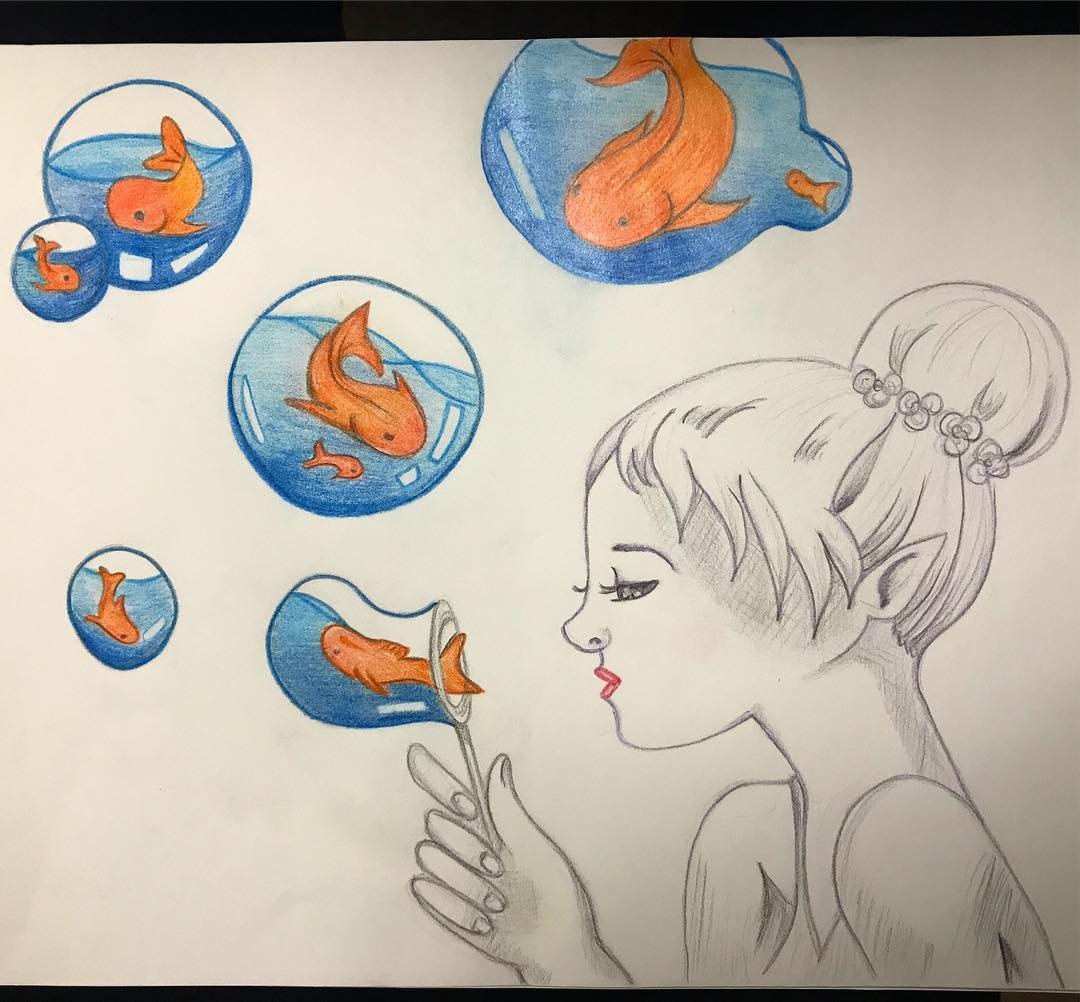This square-shaped image showcases a detailed drawing on white paper. The focal point of the illustration is a girl positioned on the left side of the image. The majority of her depiction is in black and white, save for her striking red lips which add a vivid touch of color. Her hair is elegantly styled in a bun at the back of her head, adorned with a delicate flower pattern. Her face is partially visible, revealing her left eye, ear, and nose, accentuated by her dark, defined eyebrows. Intriguingly, she appears to be holding up an object, possibly a net, with her hand, adding a sense of mystery and engagement to the artwork.